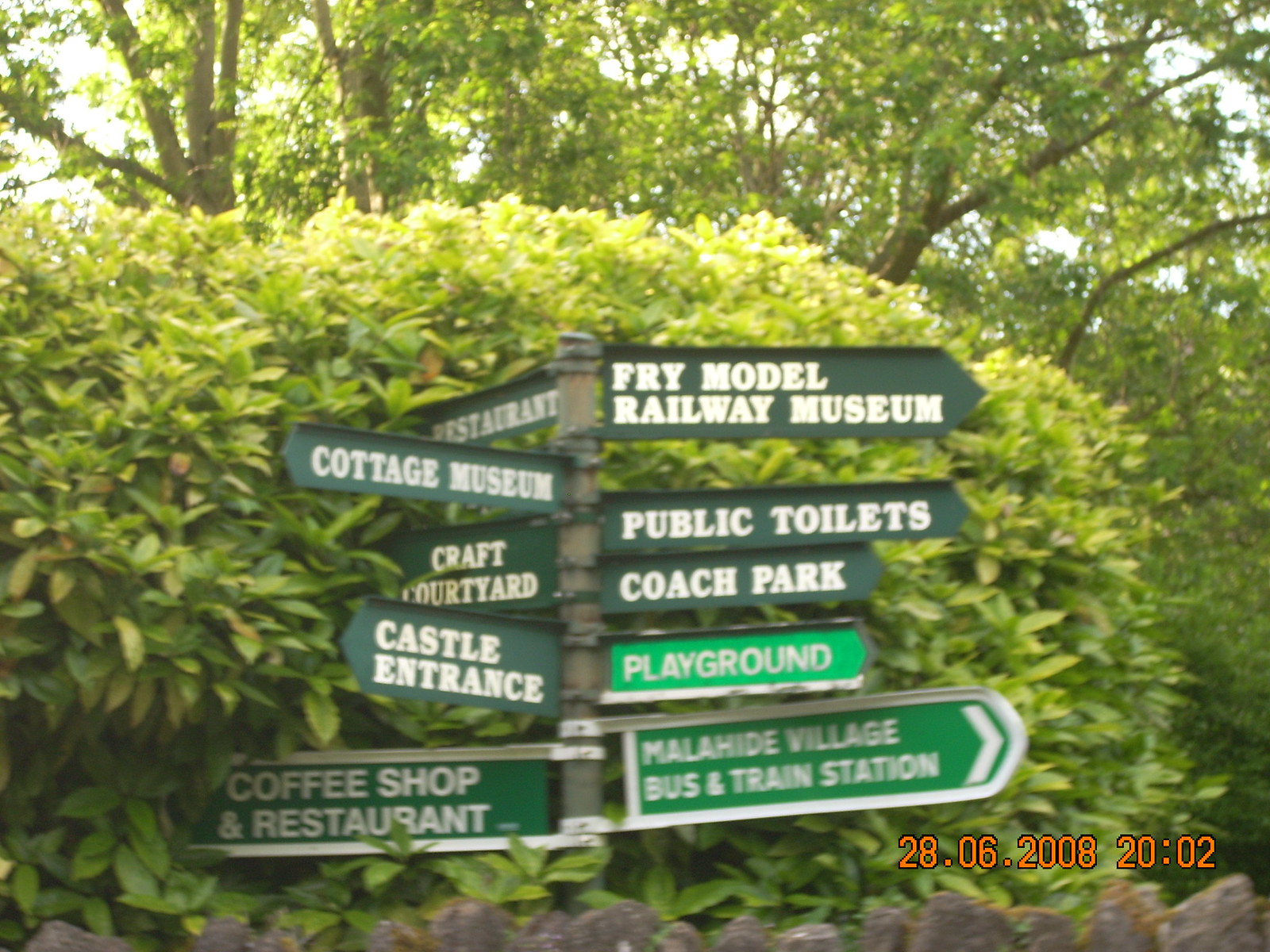The image captures a cluster of directional signs mounted on a short pole, situated outside on a sunny day. Each sign is green with white lettering, while the lower three signs feature a lighter shade of green, indicating they are newer. The signs provide directions to various locations and are shaped like arrows pointing outward. On the left side, the signs list places vertically as follows: Restaurant, Cottage Museum, Craft Courtyard, Castle Entrance, and Coffee Shop & Restaurant. The right side displays the following destinations in sequence: Fry Model Railway Museum, Public Toilets, Coach Park, Playground, Malahide Village, and Bus and Train Station. The pole appears embedded in a large green shrub with taller trees visible in the background, enhancing the natural setting. Rocks are scattered at the base of the signpost, and an orange timestamp reading "2806-2008-2002" is visible in the bottom right corner of the photo.